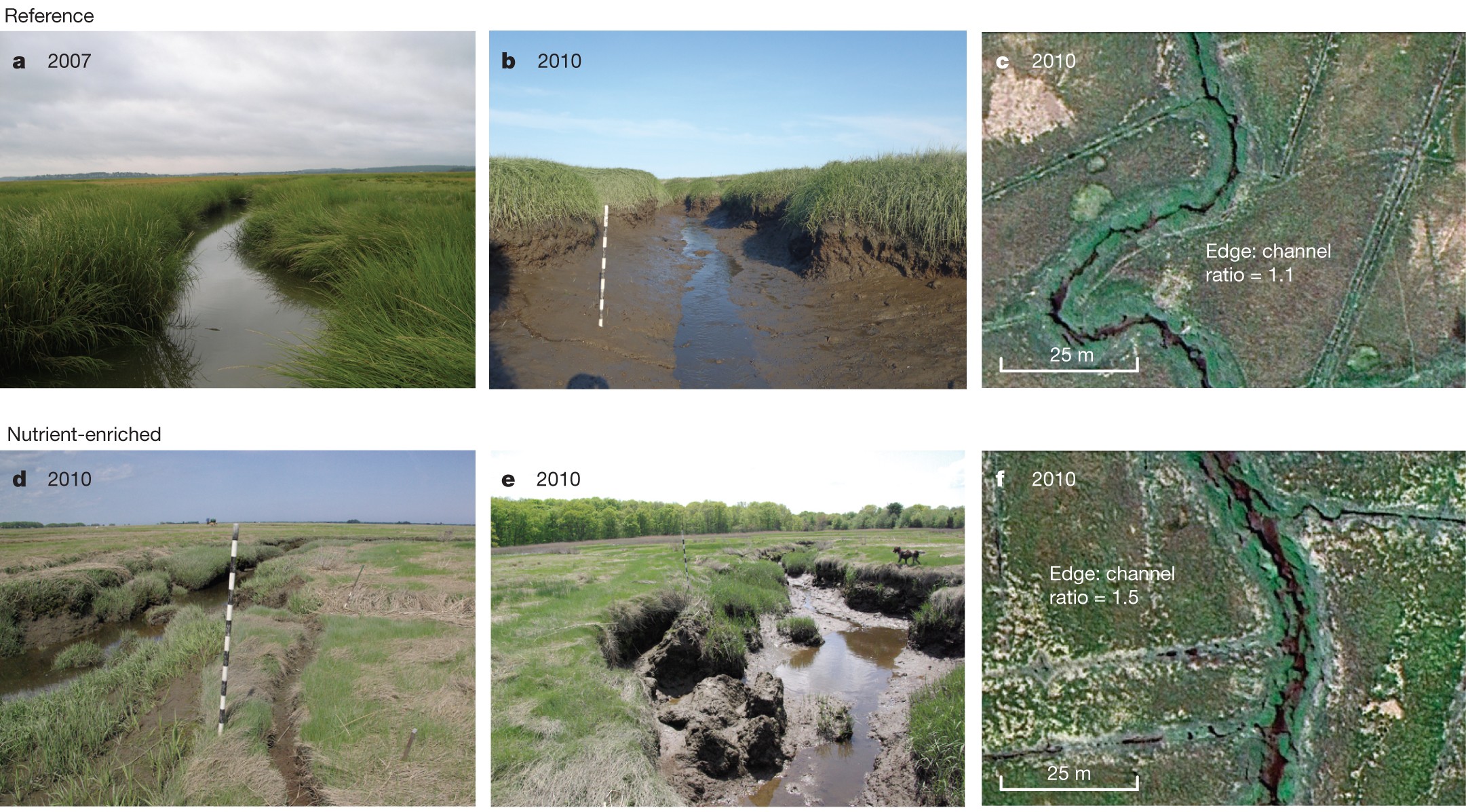This detailed image collage consists of six photographs, arranged in two rows of three, documenting changes in a river basin from 2007 to 2010. The top row is labeled "Reference" and includes: the first photo (2007) which shows a wetland area with a small creek flanked by long grass under a cloudy sky; the middle photo (B, 2010) depicts the same area with significantly reduced water levels, revealing muddy, eroded banks while grass still grows on the sides; and the third image (C, 2010) is a satellite view highlighting a curvy channel with a noted edge channel ratio of 1.1. The bottom row is labeled "Nutrient Enriched" and features: the first photo (D, 2010) showing a grassy meadow with a small creek and a black-and-white measuring pole; the middle photo (E, 2010) presents a watery, muddy landscape bordered by trees; and the final image (F, 2010) is another satellite view, this time focusing on a large trench with an edge channel ratio of 1.5. Together, these images illustrate the natural changes and significant erosion in the river basin over the years, likely serving as educational material for conservationists.